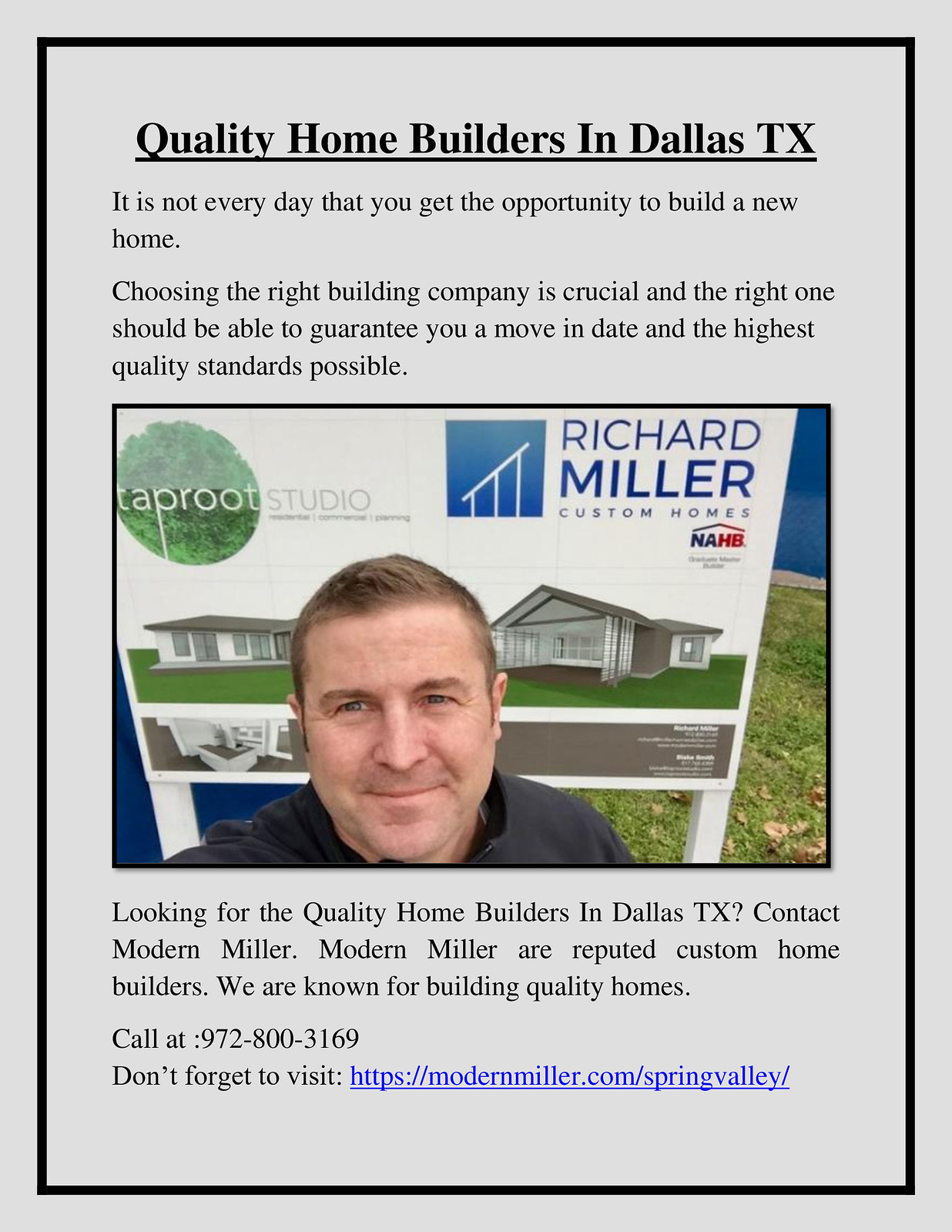This advertisement for Richard Miller Custom Homes features a light gray background with a thin black border. At the top, in bold black font and underlined, it reads "Quality Home Builders in Dallas, TX". Beneath this heading, the text continues: "It is not every day that you get the opportunity to build a new home. Choosing the right building company is crucial, and the right one should be able to guarantee you a move-in date and the highest quality standards possible."

At the center of the ad, there is a photo of a white man with short brown hair and sideburns, wearing a black sweatshirt. He is staring at the camera, and behind him is a realtor sign for Richard Miller Custom Homes, displaying images of different home models. Below the photograph, the text reads: "Looking for quality home builders in Dallas, TX? Contact Modern Miller. Modern Miller are reputed custom home builders known for building quality homes." Following this, the ad provides a contact phone number: "Call at 972-800-3169". It further encourages viewers to visit the website, displayed as a blue clickable link: "modernmiller.com/springvalley".